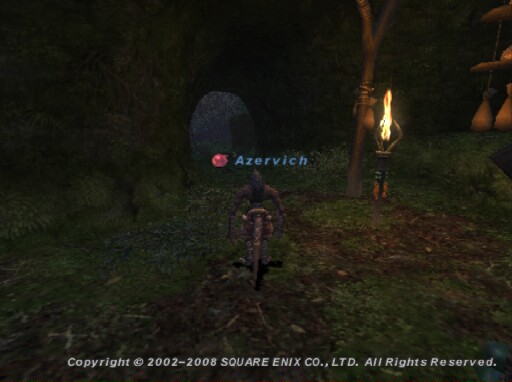In the dimly lit scene of the video game, the shadowy background frames a field or an indistinct open area. At the forefront are two intriguing characters. The first character, with a grayish hue, appears to be riding towards the observer, evoking the image of a motorcyclist. Beside him stands another character, mysteriously engulfed in flames, yet seemingly indifferent to the fire. A bare, brown tree rises starkly in the background, adding to the eerie atmosphere. To the right, a towering structure resembling a giant mushroom can be seen. Dominating the center of the image is the word "Azervich," accompanied by a red dot. Nearby, there is an ambiguous shape that could either be a tombstone or the entrance to a cave.